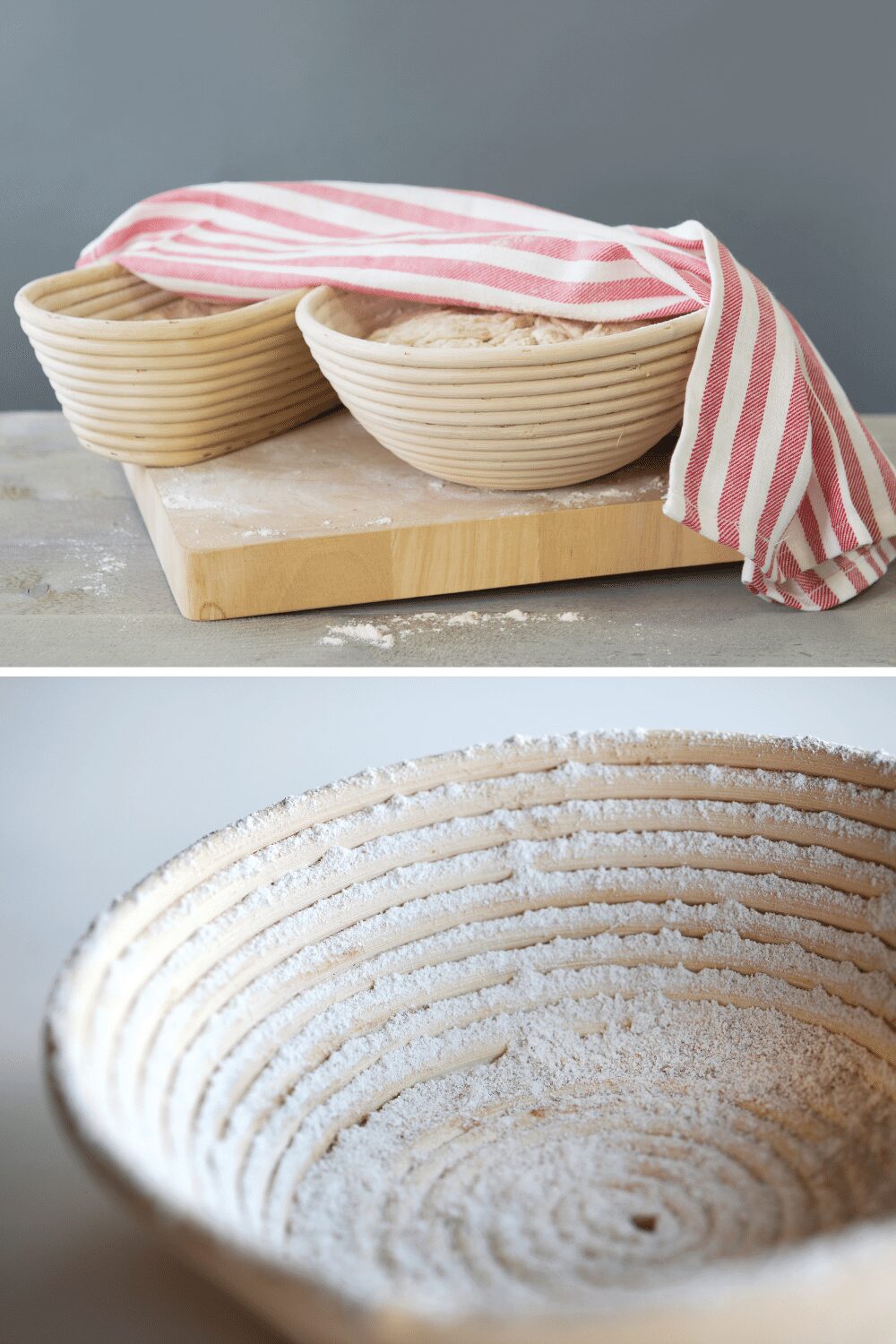This image features two photos showcasing the preparation of homemade bread. In the top photo, two proofing bowls rest on a flour-dusted wooden cutting board, which is placed on a similarly floured table. One bowl is circular, and the other is oval-shaped. A red and white striped dish towel is draped elegantly over both bowls. Inside each bowl, you can see dough in the process of proofing. In the bottom photo, a single proofing bowl is shown, filled generously with flour, ensuring the dough won't stick. This bowl has distinctive circular indents designed to imprint a unique pattern onto the bread once it's baked.